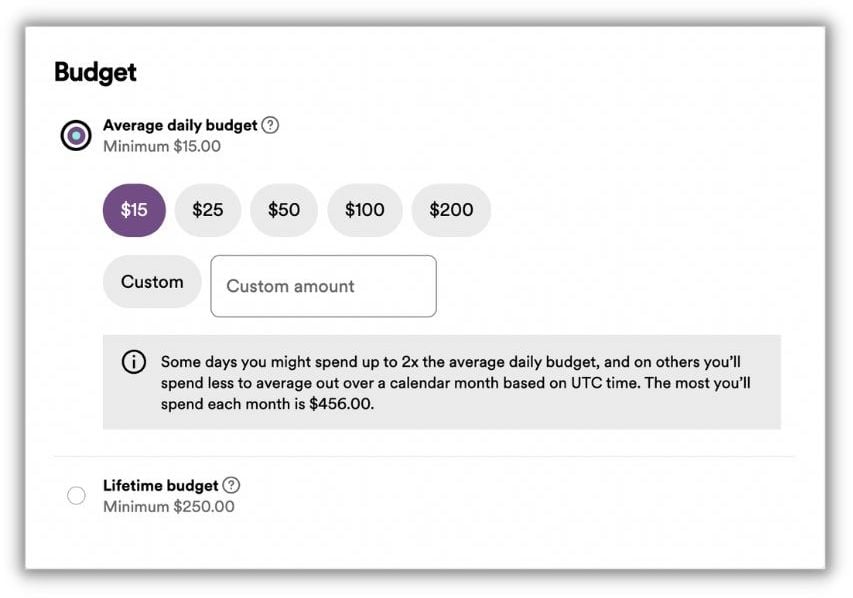The image displays a screenshot of a budgeting app, characterized by a minimalist interface. The background is white with a grey box and grey buttons featuring black text. One button stands out with purple text, indicating it's currently selected. The layout suggests this could be from either a desktop website or a partial screen capture of a mobile app.

At the top, the screen title reads "Budget" alongside a radio button option labeled "Average Daily Budget," followed by a question mark icon for additional information. The budget selection starts at a minimum of $15, offering preset choices of $15, $25, $50, $100, or $200, along with an option to enter a custom amount. Below the daily budget selection, the app informs users that daily spending might fluctuate, sometimes doubling the average daily budget, while other days may see lower expenditures. This aims to balance the spending over a calendar month, aligned to UTC time, with a cap of $456 per month based on the chosen average budget.

At the screen's bottom, there's a section labeled "Lifetime Budget," with a minimum value of $250, though this part of the interface is not selected in the screenshot. This app feature appears designed to help users set daily budgets and estimate overall spending over an extended period, such as a year.